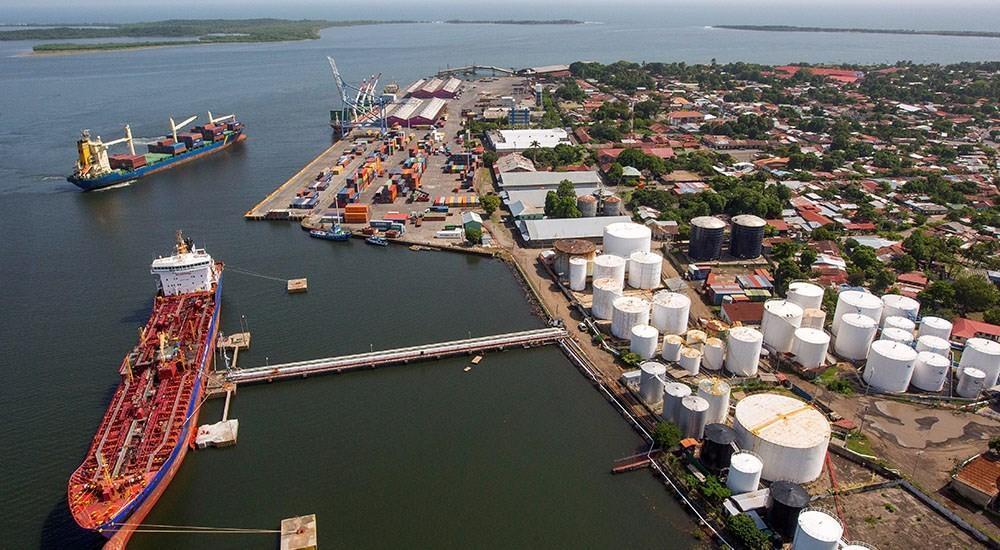This aerial photograph captures a bustling harbour port town from a high-angle perspective, as if taken from a crane or drone. On the left side of the image, a large ship is prominently docked; it features a red top deck with a blue stripe, a white bridge towards the stern, and a red hull touching the dark, almost black or deep green water. The ship is connected to the mainland by a long pier extending horizontally. Nearby, another ship with a blue bow, laden with red and blue containers and equipped with three white cranes, faces the camera but remains undocked.

In the bottom right quadrant, numerous white, cylindrical storage containers of varying sizes, resembling oversized marshmallows or candles, populate the dock area. Beyond these, stretching towards the top right, is a residential zone characterized by a grid pattern of trees and small, blurry structures, some with red or white roofs. Within the harbor's boundaries are rows of pointy-roofed buildings, colorful containers, and assorted equipment in shades of orange, blue, and other colors. Towards the top left corner, a large crane stands by the waterfront, and a ship either sailing away or approaching the port adds a dynamic element to the scene. In the far background, a couple of small islands with patches of green grass and long, irregular shapes float, framing the harbor against the sea. The image's predominant color is the dark gray-green of the water, contrasting sharply with the white structures that dot the landscape.